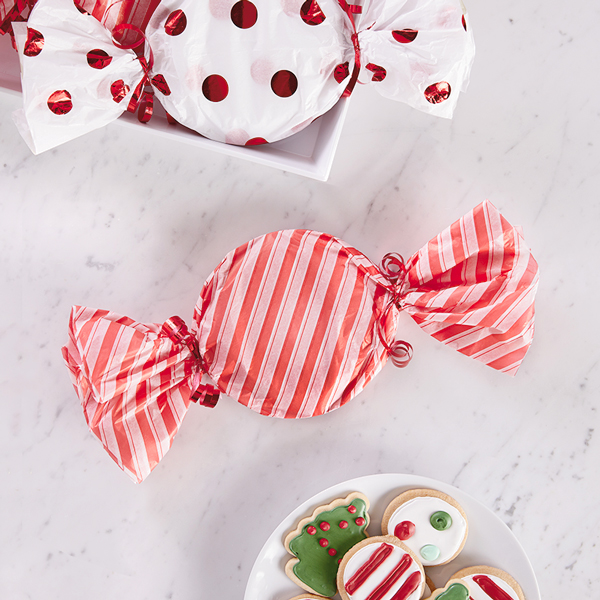On a white marble table with subtle gray speckles, a holiday-themed scene unfolds. At the top of the image, a small white tray delicately holds a large candy wrapped in white paper adorned with metallic red polka dots and tied with matching red string. Directly below it, a similarly wrapped larger candy features diagonal red and white stripes, secured with red ribbons at the ends, creating the appearance of oversized Christmas peppermint candies. This candy rests freely on the table. At the bottom of the image, a white plate showcases a delightful assortment of Christmas cookies. The cookies are frosted in white, with one shaped like a Christmas tree, decorated with green icing and red dots. Among the assortment are circular cookies, one with white frosting and red stripes, and another with white frosting and colorful dots in green, red, and light blue. The entire scene is bathed in bright light, highlighting the festive details and evoking a cheerful holiday spirit.